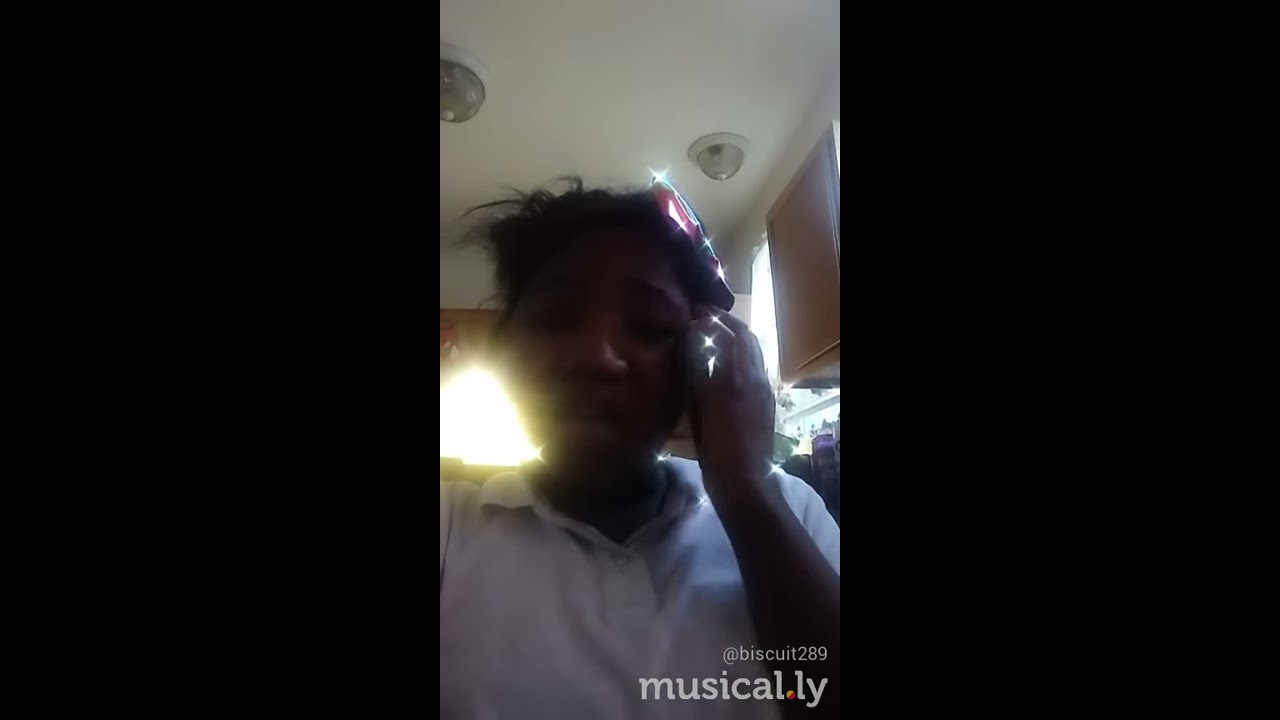The image is a vertical still taken from a short video, likely on TikTok, given its smartphone-like dimensions with large black borders on either side. At the bottom of the frame, there's a username "@biscuit289" followed by the text "musical.ly," suggesting it might be the platform's URL. In the image itself, a young black woman with black curly hair, wearing a white polo shirt, is standing in what appears to be a kitchen. She has her hand up to her ear, and there is a pink and teal sparkling accessory in her hair on the right side. The environment features a white ceiling with light fixtures, light brown cabinets on the right, and sunlight streaming through a window behind her on the left, creating a slightly out-of-focus effect. Another window on the right side, partially blocked by a cabinet, also lets in some light, which illuminates potential plants on the windowsill.